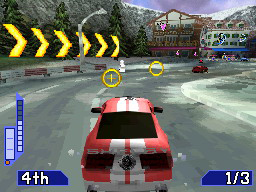A vibrant screenshot from a racing video game features a stylized red car with a prominent white stripe curving sharply to the right. The car, adorned with an indistinguishable emblem and obscure lettering that appears to spell 'shady', is mid-race. In the upper left corner, the screen displays 'fourth' and 'one third' on the right, likely indicating the player's position and lap progress. The left side of the screen is lined with yellow arrows pointing to the right, signaling the impending right-hand turn. Ahead of the main car, another vehicle can be seen, and there are two overlapping circles and a cross symbol on the left, potentially indicating a gameplay feature related to targeting or interaction. The game's detailed graphics and interface create an immersive racing environment.